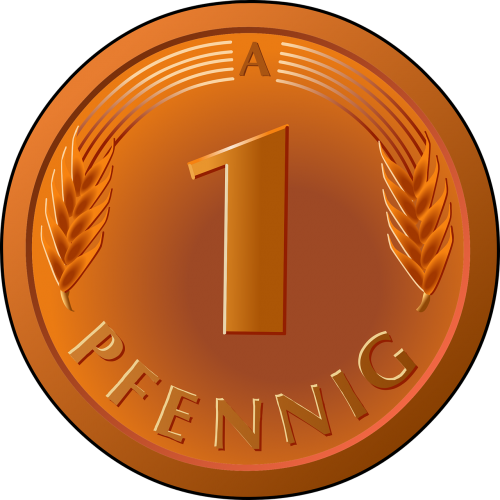The image features a digitally created, circular coin set against a white background, presented in a cartoon style. Dominating nearly the entire frame, the coin sports a bronze or orange hue with shades of black, brown, brass, and gold. Central to the coin's design is a large number "1," flanked on either side by elongated barley-wheat motifs. At the top, the letter "A" is prominently displayed, accompanied by curved lines extending towards the wheat designs. The bottom of the coin reads "PFENNIG," indicating its type. Black lines outline the coin and its inner circle, giving it a detailed and shaded appearance. Overall, this illustration resembles an oversized penny or a European currency mock-up.